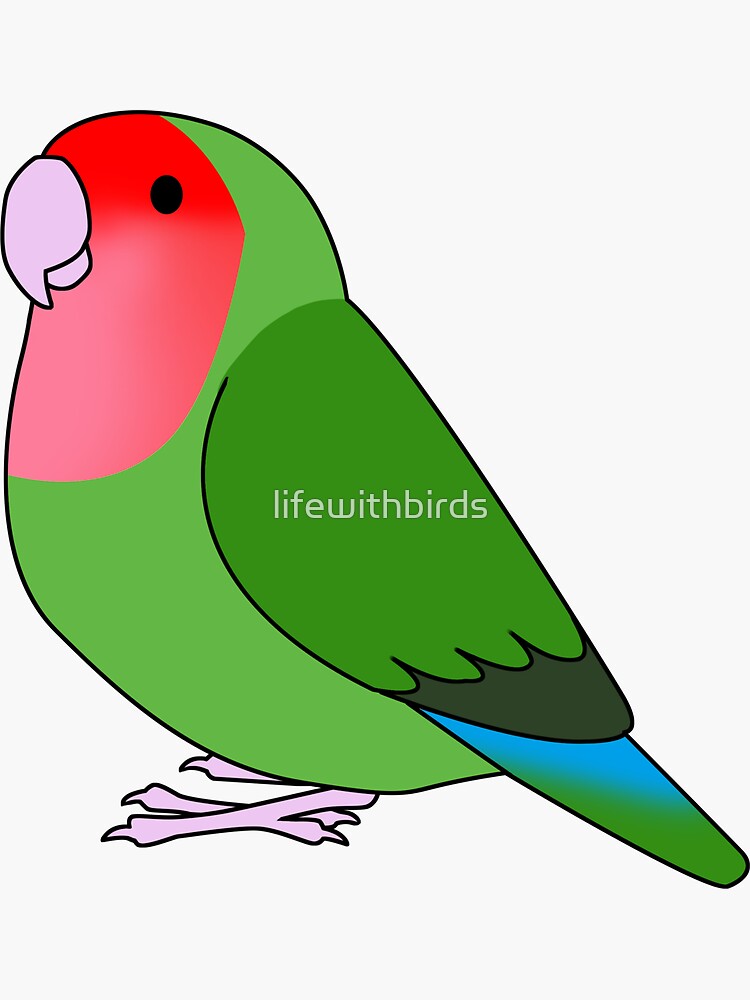This vertical image features a detailed and colorful illustration of a parrot, set against a very light gray background. The parrot, which appears to be the focal point of an ad: "Life with Birds" written in small, yellow lowercase letters across its wing. The parrot is primarily green, with its body and wings depicted in various shades of green and darker green. The tips of its wings are black, and there is a variegated blue coloring subtly peeking from underneath the wings near the tail. The parrot's tail is a darker green but also includes touches of blue at the top. Its face and throat are strikingly red, contrasting with its black eyes and pointed pink beak. The parrot has pink legs and feet, with three toes visible. The bird is oriented with its head facing towards the top left of the image and its tail towards the bottom right. The overall simplicity of the design, combined with some shading and detail, gives it a clean, almost computer-colored appearance.